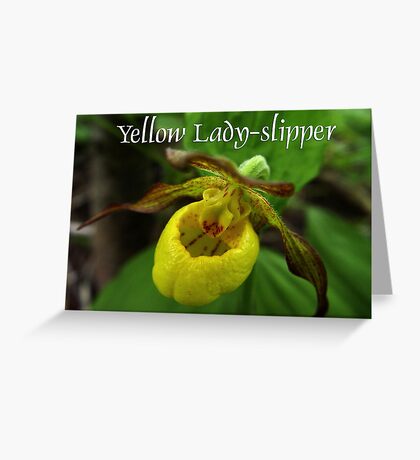This image features a card with a white background, showcasing a detailed photograph of a Yellow Lady Slipper plant. The card flips up rather than from left to right, indicated by the gray shaded backside visible on the right. Centered on the card is the plant’s name, "Yellow Lady Slipper," written in white text at the top. Below the text, the vibrant plant is depicted with downward-tilted leaves, three prominently coming towards the viewer. Beneath these leaves, there are tiny green sprout-like objects, leading to a distinctive yellow, bowl-shaped part of the flower, known for containing numerous black seeds. The yellow section, which gives the plant its name, is adorned with red dots on the inside and outside of the petals. This all stands out against a mostly green and dark backdrop, suggesting the photograph was taken in a dense, natural setting like a forest.